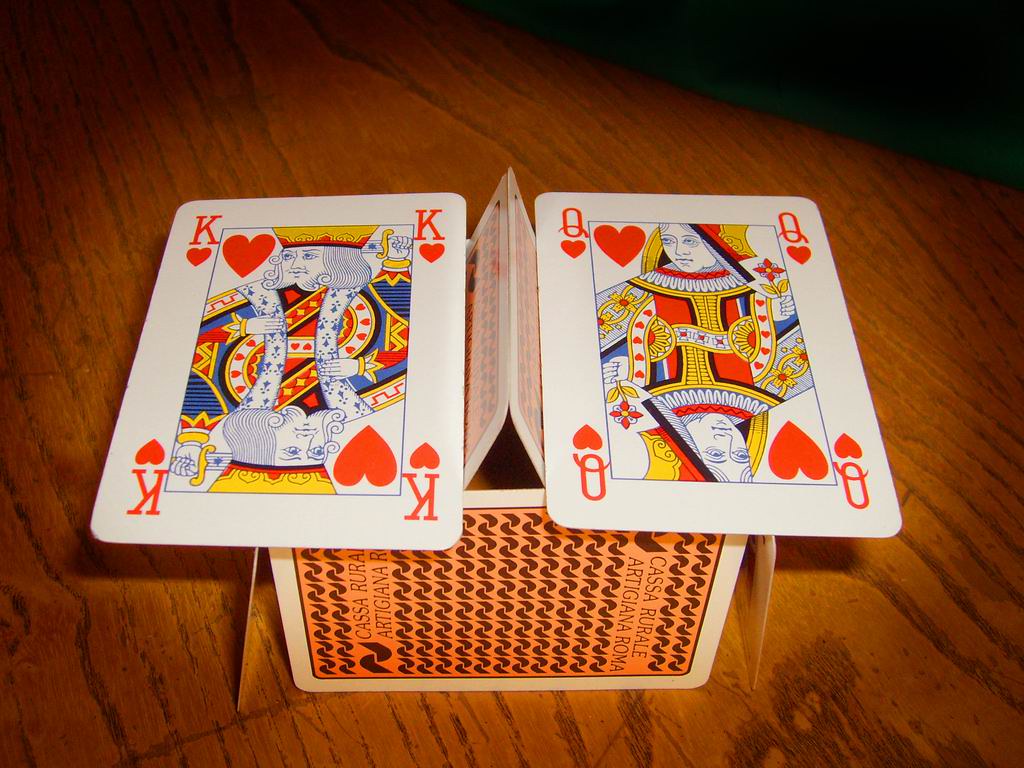A beautifully crafted structure of playing cards sits upon a cherry wood surface, showcasing intricate grain lines. The cards are meticulously arranged to resemble a small building, featuring a pointed roof. On the left side, the King of Hearts card is prominently displayed, bearing the traditional imagery of a crowned king, mirrored by its inverted twin below. To the left of the king, the Queen of Hearts stands gracefully, holding a delicate flower. The back of one of the cards is partially visible, adorned with ornate swirly shapes and inscribed with the text "Casa Rurale Artigiana Roma." The entire scene captures a blend of elegance and playfulness, set against the rich, reddish-brown backdrop of the polished wood.